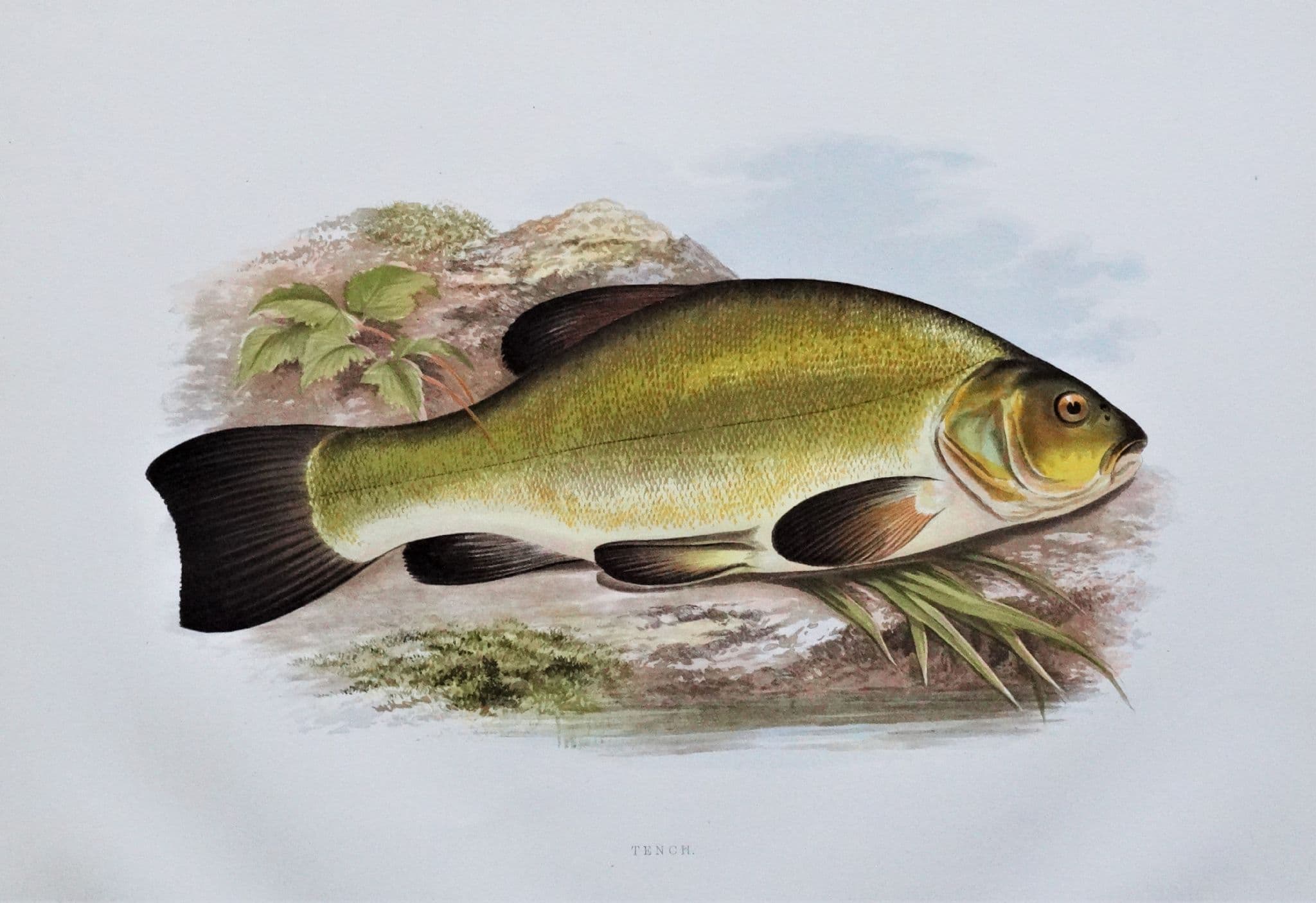This image is a colored painting of a horizontally-placed fish on a whitish-grayish background. The fish is labeled with small, unclear letters at the bottom that appear to spell "T-E-N-C-H," which is likely the name of the fish. The fish itself exhibits a goldish-grayish color with a white belly. Its fins are predominantly black, with some gray and light brown shading, especially on the fin closest to the head. The eyes are a striking goldish-yellow color, contributing to a perpetually frowning expression.

Surrounding the fish, the background features green leaves, a branch, and elements suggestive of a mountain and lake setting, while a couple of planks appear beneath and near the fish. Additionally, there is a stone ground-like structure partially visible beneath the fish. The image portrays the fish with a blend of green and yellow tints on its body, emphasizing its natural aquatic environment.